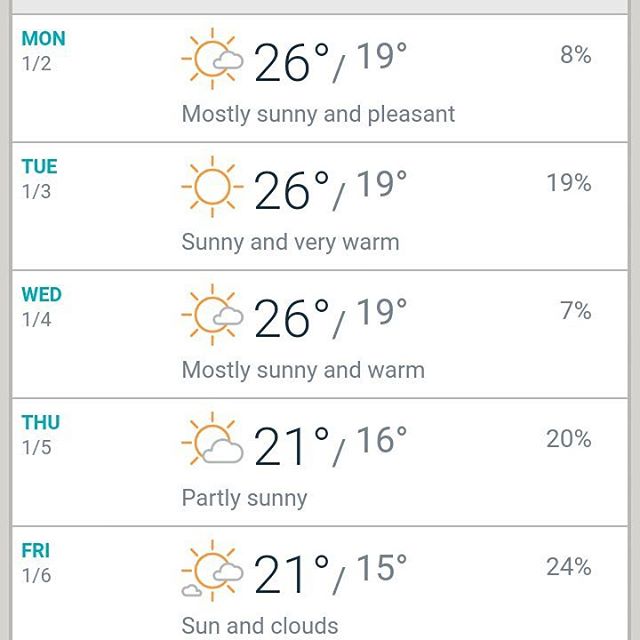The image presents a detailed weather forecast for the weekdays, beginning with Monday and ending with Friday. The forecast is divided into five sections, with gray borders framing the top of the image. Each day of the week is marked in blue letters starting from the top left corner with "MON" for Monday, followed by the dates and weather information sequentially down the image. 

- **Monday (MON 1/2)**: Illustrated with a sun partially obscured by a small cloud. The forecast notes a high of 26°C and a low of 19°C, with an 8% chance of precipitation. The description reads "mostly sunny and pleasant."
  
- **Tuesday (TUE 1/3)**: Showcases a sun without any clouds. The temperature is forecasted at 26°C/19°C. The weather is described as "sunny and very warm," and a 19% chance of rain is noted.

- **Wednesday (WED 1/4)**: Depicts a sun partially obscured by a small cloud. Temperatures remain steady at 26°C/19°C, with a 7% chance of rain. It is described as "mostly sunny and warm."

- **Thursday (THU 1/5)**: Features a sun heavily obscured by a large cloud. The temperature drops to 21°C/16°C, and there is a 20% chance of rain.

- **Friday (FRI 1/6)**: Shows a sun flanked by a small cloud on the bottom left. The temperatures are a high of 21°C and a low of 15°C, with a 24% chance of rain. The description reads "sun and clouds."

Overall, the image offers a clear and concise visual representation of the upcoming week's weather, highlighting daily temperatures, weather conditions, and precipitation chances.